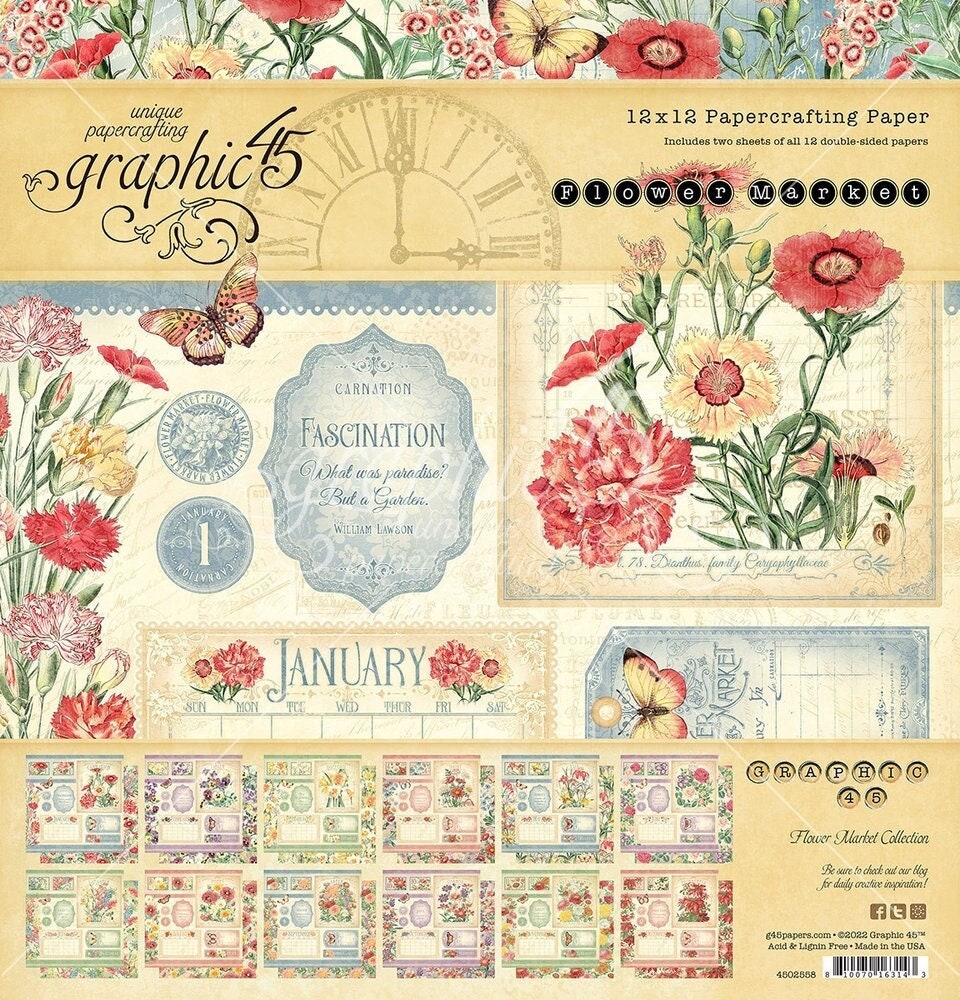This is a vibrant and detailed color photograph advertising the "Graphic 45 Flower Market Collection" of 12x12 double-sided crafting paper. The image is a top-down view of an unopened package featuring multiple sheets of unique floral and butterfly designs, organized by the months of the year, from January through December. Central to the image are vivid illustrations of flowers in various pastel shades—red, yellow, pink—alongside butterflies, enhancing its colorful appeal. The packaging prominently displays "Unique Paper Crafting, Graphic 45," along with the "Flower Market" branding. Additionally, a light blue crest with the words "fascination carnation" adds a touch of elegance. At the top of the page, and scattered throughout, more floral graphics and butterflies can be found, heightening the overall decorative theme. The advertisement also highlights that the product is "Made in the USA" and encourages viewers to visit their blog for daily creative inspiration. Social media links and a barcode are visible at the bottom, indicating the commercial and interactive aspects of the product.